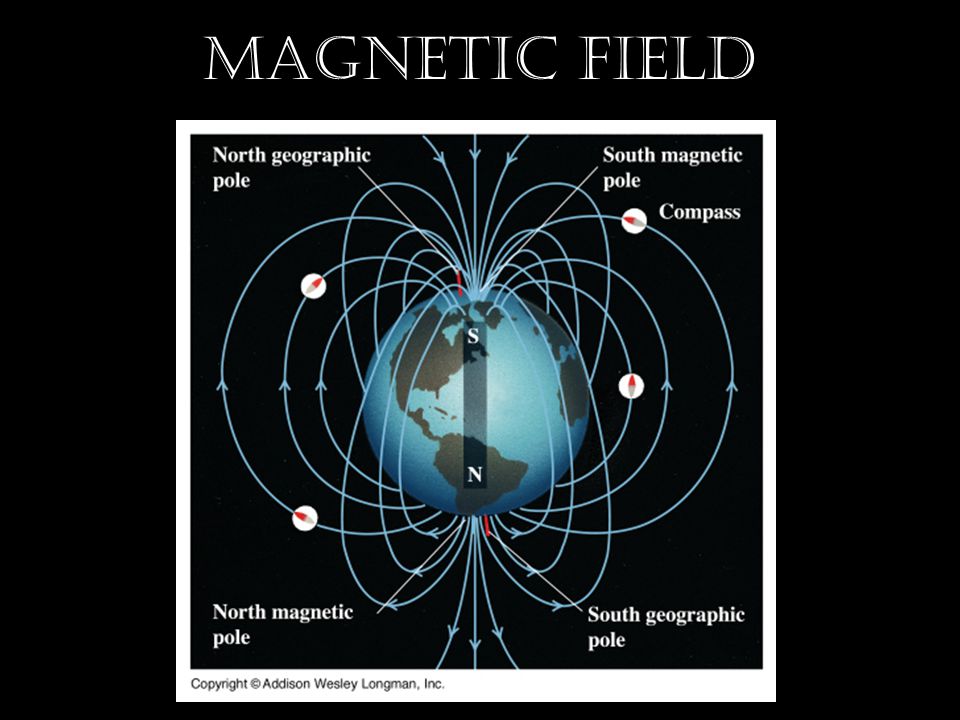This educational poster, with a black background and a white border, prominently features the title "MAGNETIC FIELD" at the top in bold white capital letters. Inside the bordered area, a detailed illustration of the Earth is displayed, primarily showcasing the Americas with parts of Europe and Africa visible on the right side. The globe is depicted in blue, with continents outlined in black. The illustration aims to explain the Earth's magnetic field, as indicated by multiple curved blue lines that loop from the north geographic pole to the south geographic pole and from the north magnetic pole to the south magnetic pole, demonstrating their interactions. Various labels in white text point to specific areas: "North Geographic Pole," "South Magnetic Pole," "Compass," "North Magnetic Pole," and "South Geographic Pole." These labels help illustrate the functioning of a compass and the positions of the magnetic poles. At the bottom left corner of the white border, "© Addison-Wesley-Longman, Inc." is written in small black letters, indicating the copyright holder.